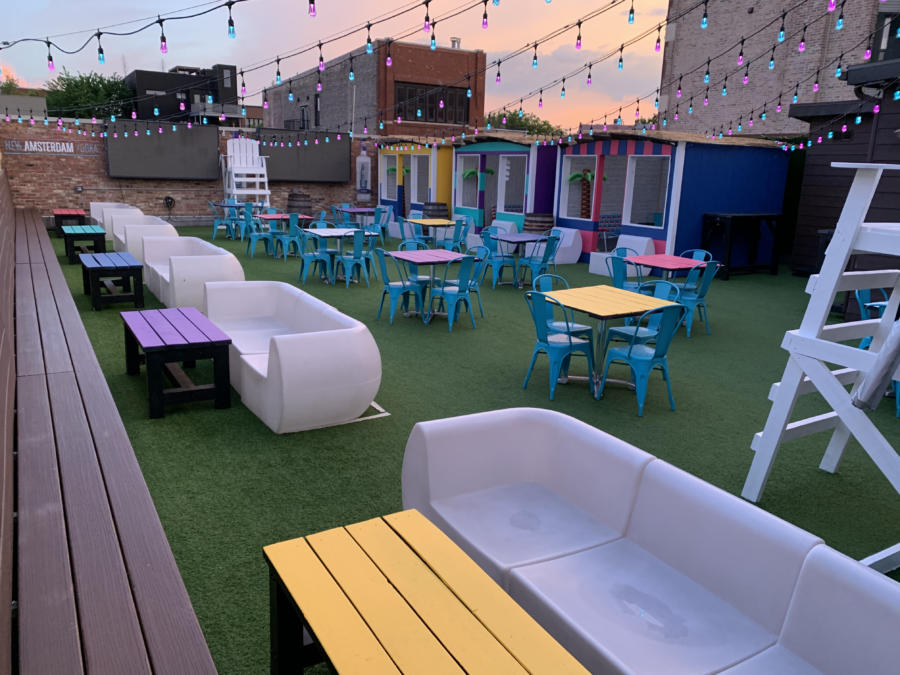The image depicts a vibrant outdoor party venue or social gathering area, likely situated in an urban environment. The scene is characterized by an expanse of very green astroturf, simulating a lush lawn. This synthetic grass stretches beneath a colorful array of furniture and decorations, creating a lively, welcoming atmosphere.

In the foreground, there are numerous white plastic settees arranged in a cozy, lounge-like manner, each accented with a brightly colored wooden coffee table—colors such as red, blue, purple, lighter purple, yellow, and pink stand out. The seating arrangement extends to include both benches and small plastic couches that offer ample spots for socializing.

Scattered throughout the area are multiple square tables, each paired with four chairs. The tables feature various vivid tabletop colors: yellow, blue, orange, purple, and pink, complemented by blue and green plastic chairs. These seating arrangements are spread out, fostering a communal vibe.

Towards the back of the venue, there are three small huts or sheds, which might be used for food service or other activities. These huts are painted in cheerful tropical hues like yellow, blue, and purple, with one even featuring red and blue stripes, enhancing the festive feel of the venue.

Overhead, string lights crisscross the sky, adding both charm and illumination. The lights predominantly feature colors like turquoise, purple, pink, and blue in rotating patterns. The entire setting is framed by a brick wall bearing a sign that reads "New Amsterdam," adding a touch of urban authenticity. This brickwork backdrop includes a mix of tan, brown, and other earthen shades, and is punctuated by a couple of TVs, currently turned off.

The sky includes hues of sunset or early morning light, adding a soft natural gradient to the scene. Buildings with varied facades—black, red brick, off-white brick—peek above the wall, indicating that this lively venue is likely on a rooftop or in an elevated urban space. Overall, the image captures a colorful, detailed, and inviting setting perfect for social gatherings and entertainment.